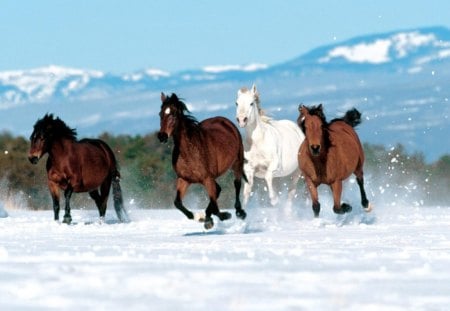In this vivid daytime photograph, four horses gallop through a snow-covered field, kicking up a flurry of white powder. The central figures, positioned prominently in the image, include two dark brown horses with black manes and tails, another dark brown horse with white markings on its head, and a striking all-white horse with a tan mane and pink nose. To the back of this dynamic scene, a snow-capped mountain rises majestically against a vibrant blue sky, flanked by a lush line of green-leaved trees. This captivating and energetic moment encapsulates the essence of wild beauty amidst a winter landscape.